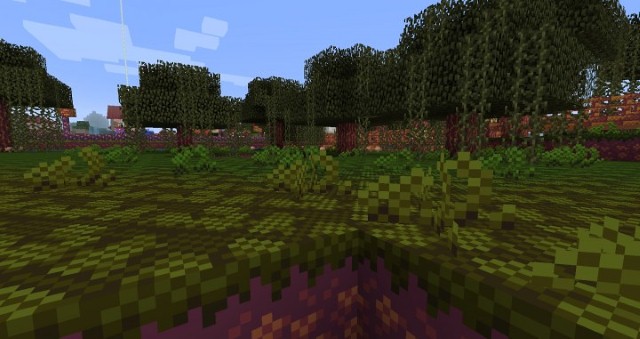In this image, we see a detailed Minecraft scene that captures the essence of the popular video game. At the bottom of the image, there's a distinctive strip of purple ground, which stands out against the predominantly green terrain above it. The green ground is interspersed with light brown shading, adding texture and depth, and transitions to darker green towards the background.

The landscape features cube and rectangular-shaped trees with brown trunks and dark green foliage. In the distance, some square-like shapes in brown and green are visible, adding to the scene's complexity. The sky above is a light blue, with several white, flat platforms scattered along the left-hand side, resembling clouds or elevated structures. This detailed depiction captures the characteristic blocky aesthetic of Minecraft, blending vibrant colors and geometric shapes.